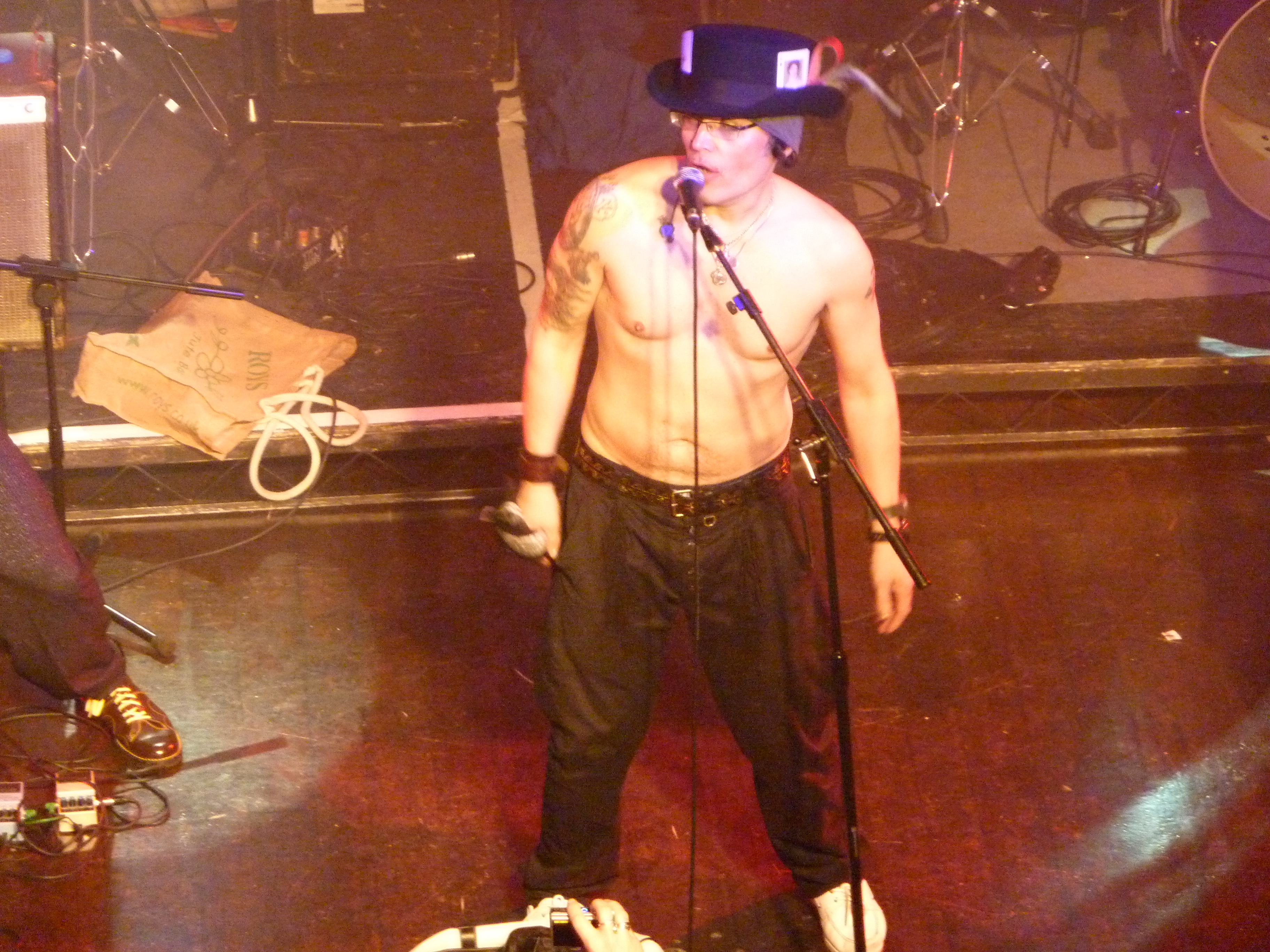The photograph, though of lower quality indicating its age, captures a shirtless man on a dark wooden stage, standing close to a microphone. He wears black trousers with a brown belt and a short, dark purple top hat adorned with a couple of cards and a decorative banner. His arms rest by his sides, revealing tattoos on his left shoulder, and he sports rectangular glasses and wristbands on both wrists. His body faces forward, but his head is turned towards the left, engaging with something or someone out of the frame. The microphone has a black body with a silver head, positioned near his mouth to the right. The picture, taken from a higher angle, shows scattered stage props including metal stands, electrical cables, and a bag in the background. On the left side of the image, another person's leg in dark pants is visible, while in the bottom right, a black leather shoe and some foot pedals can be seen. Additionally, two hands are visible at the bottom center of the image, alongside the bright stage lights casting a glow over the scene.